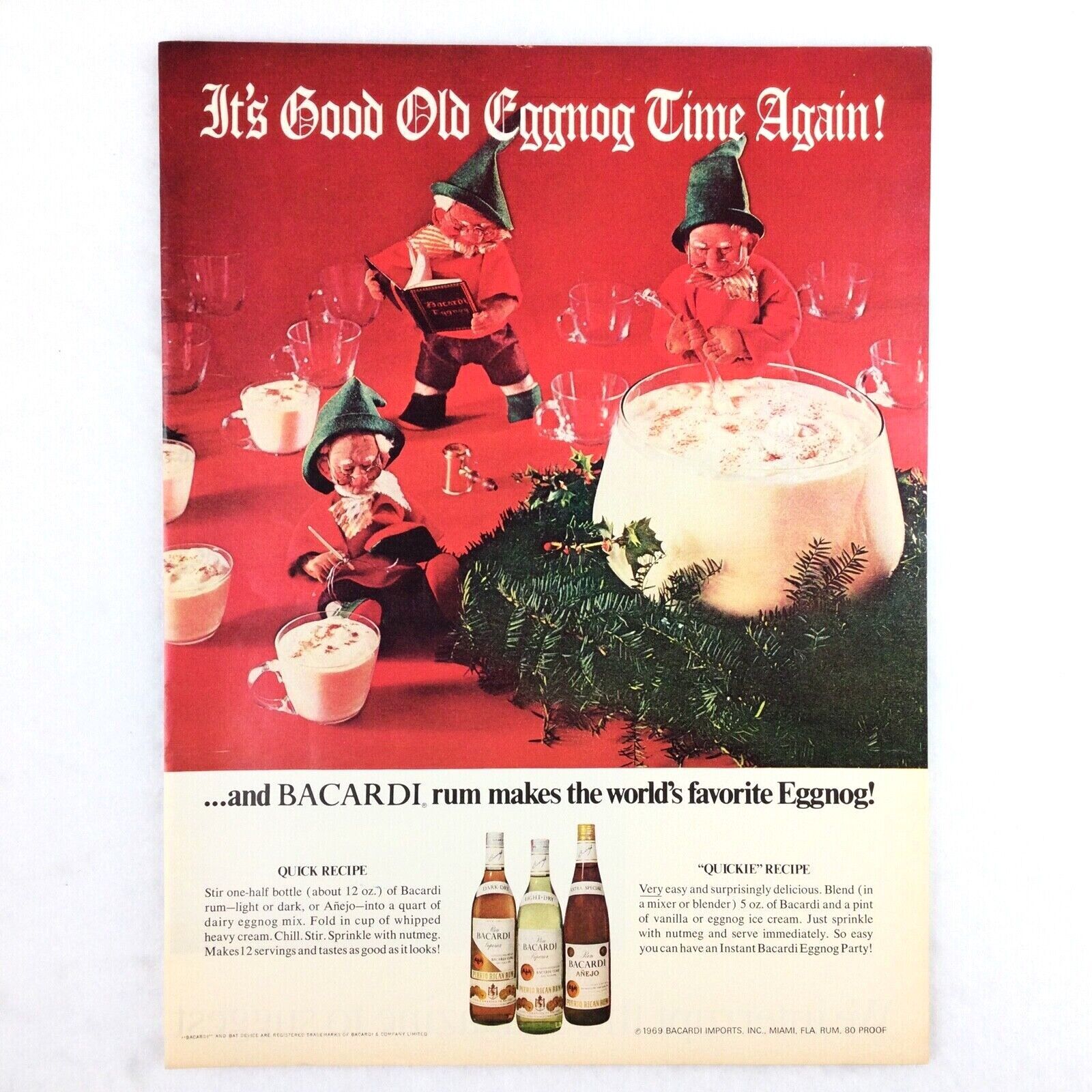This vintage 1969 Bacardi Rum advertisement features a festive scene with three Santa's Workshop-type elves in red smocks and green hats. They are gathered around a large glass of eggnog, filling small mugs with the creamy drink. The scene is set against a vibrant red background, with a Christmas wreath adding to the holiday spirit. At the top, in classic Old English font, the text exclaims, "It's good old eggnog time again." Below, on a beige background, the message continues with, "And Bacardi Rum makes the world's favorite eggnog," accompanied by images of three Bacardi bottles—each a different variety. To the left, a detailed recipe instructs readers to mix half a bottle of Bacardi rum with a quart of dairy eggnog mix and whip in heavy cream, suggesting serving with a sprinkle of nutmeg. On the right, an easier "quickie recipe" recommends blending rum with vanilla or eggnog ice cream. Overall, the advertisement exudes vintage holiday charm, offering festive recipes for a Bacardi eggnog party.